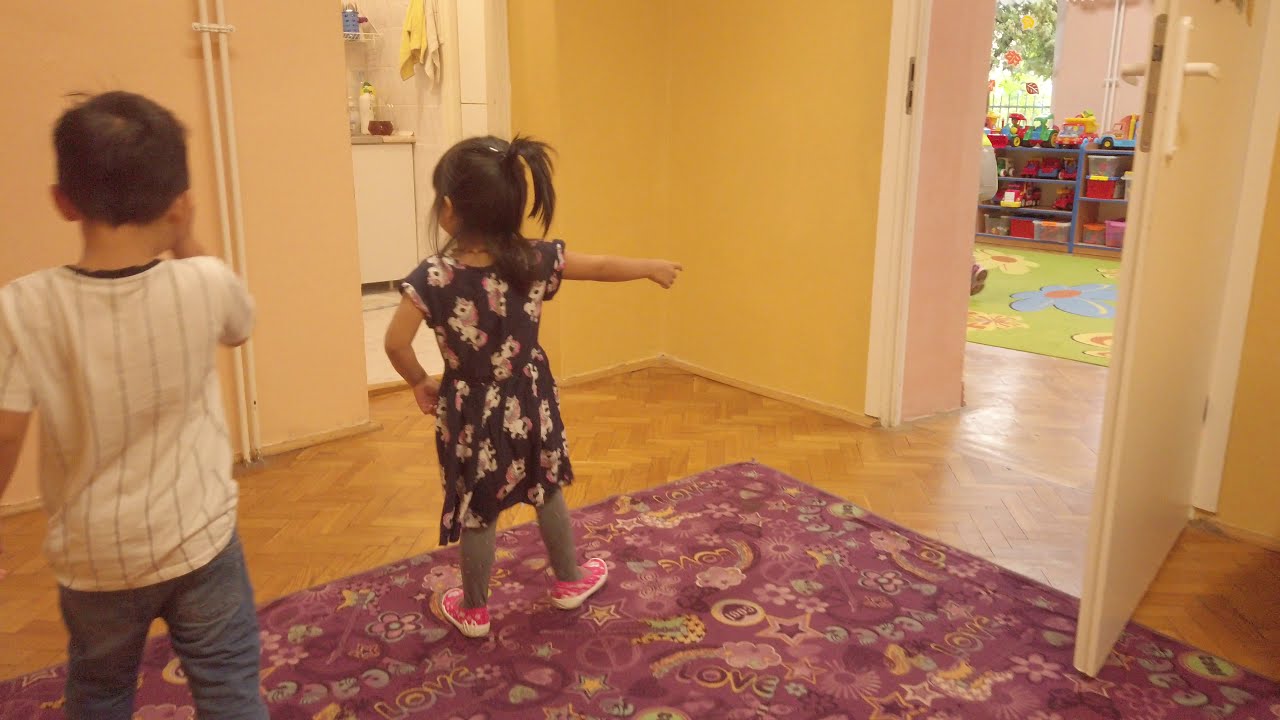This photograph captures a moment inside what appears to be a home, though it could also be a school or daycare. In the center-left of the image, two young children with dark hair are standing on a purple rug adorned with stars, peace signs, the word "love", rainbows, and clouds, which lies on a brown hardwood floor. Their backs are to the camera, and they appear to be around five to seven years old. On the left, the boy is dressed in blue jeans and a white shirt with thin black vertical stripes. To his side, the girl wears a black dress featuring a floral and unicorn print, pink shoes, gray leggings, and her hair pulled into a ponytail. She points toward a room to her right, which has an open white door with a yellow handle. Inside this room, there's a colorful green rug with large yellow and blue flowers and shelves filled with various plastic toys. Beyond the children, there’s also a glimpse of a kitchen area with white lower cabinets and shelves holding containers, framed against yellow walls. This setting suggests a lively and playful environment for the children.